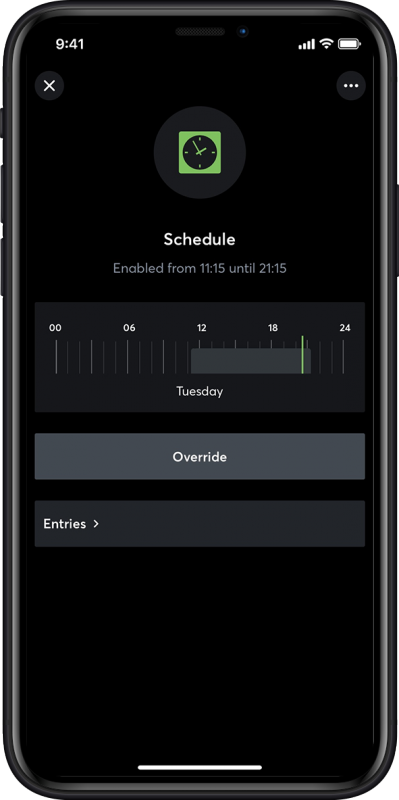In this detailed image, we see a cell phone with a black outline and a gray internal line surrounding a black screen. On the left side of the phone, there are three buttons: a short one and two longer ones. On the right edge, there is a long and flat button. 

In the top left corner of the screen, the time "9:41" is displayed in white font. On the top right, there are icons for the Wi-Fi signal and battery status. Below these, on the left side, there is a white "X" symbol inside a gray circle. On the right side, within a gray circle, there are three dots. 

In the middle of the screen, there is a slightly darker gray circle featuring a square clock with long and shorthand. Below this clock, in the center, is the word "Schedule" in white font. Underneath, in gray font, it states "Enabled from 11:15 until 21:15." 

A gray bar below this has a box featuring the numbers "00, 06, 12, 18, and 24" with gray lines in between. Between the numbers "12" and "just past 18," the bar turns a darker gray. 

Under this section, "Tuesday" is written in white font. The next gray box below is darker and contains the word "Override" in white font in the center. 

In the box below that, which is slightly darker gray, the word "Entries" is written in white font on the left, with a white arrow pointing to the right next to it. At the very bottom of the screen, there is a thick white line in the center.